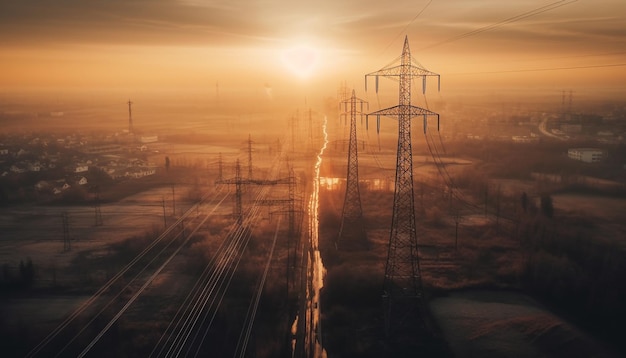The image depicts a vast, stark scene of an industrialized field bathed in the hues of sunset, with varying shades of oranges, browns, and beiges. The setting sun, partially obscured by clouds, casts a golden and yellow light over the entire landscape, imparting an almost surreal night-like quality to the image. Central to the composition is a thin, bright streak reminiscent of lightning or a waterway reflecting sunlight, stretching from the distant sun to the foreground, adding a dynamic element to the scene.

On the left, there is a road accompanied by train tracks, possibly leading to a neighborhood with a cluster of buildings and houses. This area is lined with tall electrical towers and power lines, emphasizing the industrial nature of the setting. To the right, alongside smaller ponds of water, similar tall powerline towers are visible, further framing the barren landscape.

The overall mood of the image is one of desolation and harsh beauty, where industrial elements blend seamlessly with natural features under the striking evening sky. The pervasive reddish-brown tint and the light haze give the scene an almost frosty appearance, adding to its bleak yet captivating atmosphere.